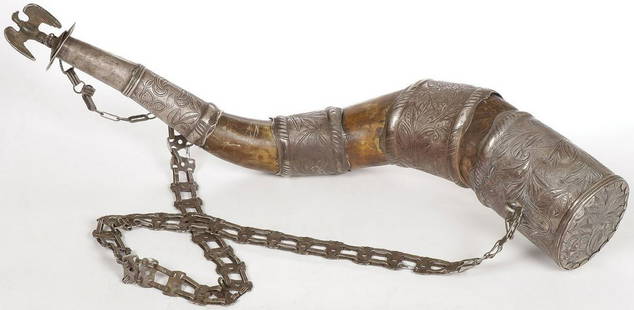This photograph features a highly intricate and likely antique object that could be a drinking horn or an old gunpowder storage device, possibly from the Civil War era or earlier. The piece is made of a bronzish-colored metal with significant tarnishing, complemented by decorative, engraved silver rings and carvings along its shaft. A chain, ranging from dark gray to light silver, connects from the wider top end, adorned with elaborate engravings and a cap, down to the narrower tip, which is fitted with a cork topped by a small figurine resembling an American Eagle. The entire object shows signs of age but remains in remarkably good condition, highlighting its historical significance and craftsmanship.